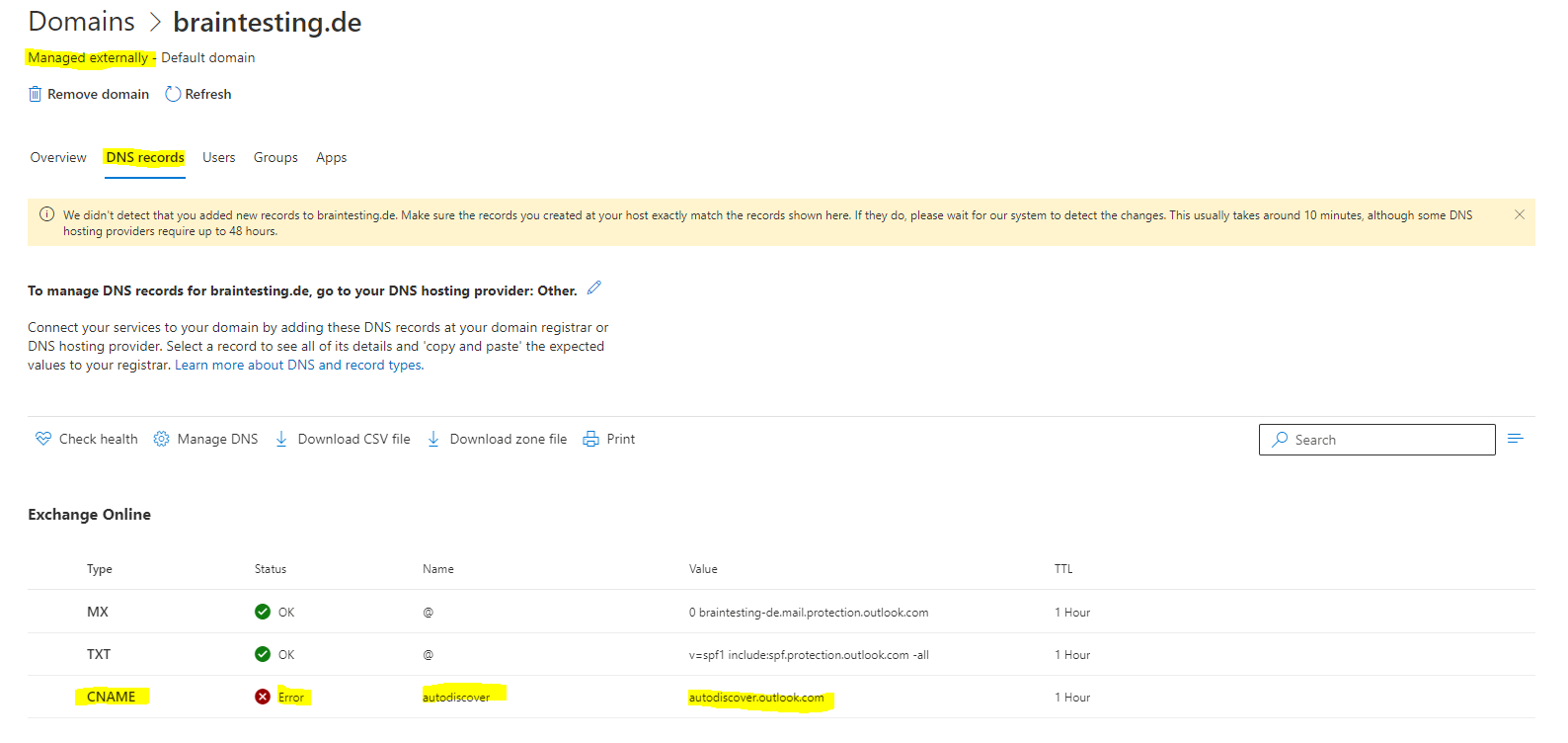The image depicts a white background filled with an assortment of textual elements, mostly in black and gray fonts. The content is slightly blurred and zoomed out, making the text hard to discern clearly. At the top of the image, the word "Domains" is written in a standard font, followed by a bolder text stating "braintesting.de." Below this header, it mentions "managed externally" and "default domain," with "managed externally" highlighted in yellow.

Further down, several sections and labels are listed in black text, including "Overview," "DNS Records" (highlighted in yellow and underlined in blue), "Users," "Groups," and "Apps." There is also a prominent red text box containing some blurred black text and a black X icon inside it.

Underneath the red text box, the text reads: "To manage DNS records for braintesting.de, go to your DNS hosting provider," next to the word "other" which is accompanied by the image of a small pencil.

At the bottom portion of the page, three circles are present: two green circles with white check marks inside them labeled "OK," and one red circle with a white X labeled "Error."